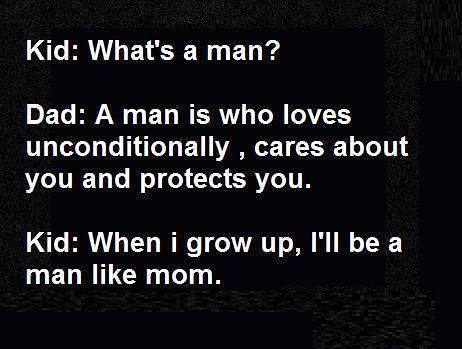The image features a predominantly black background with a slightly staticky texture in shades of dark gray around the edges—primarily at the top, left-hand side, bottom, and right, creating a subtle outline. Centered on the background is a conversation in white text, likely captured from a computer screen. The dialogue begins with "Kid:" followed by "What's a man?". Next, labeled "Dad:", the response reads, "A man is who loves unconditionally, cares about you and protects you." The exchange concludes with "Kid:" saying, "When I grow up, I'll be a man like mom." This text, formatted with uppercase for "Kid" and "Dad" and lowercase for the second "I" in the kid's last line, humorously highlights that qualities attributed to men also apply to women, suggesting a playful jab at traditional gender roles. This type of nuanced and relatable humor is often shared on social media.